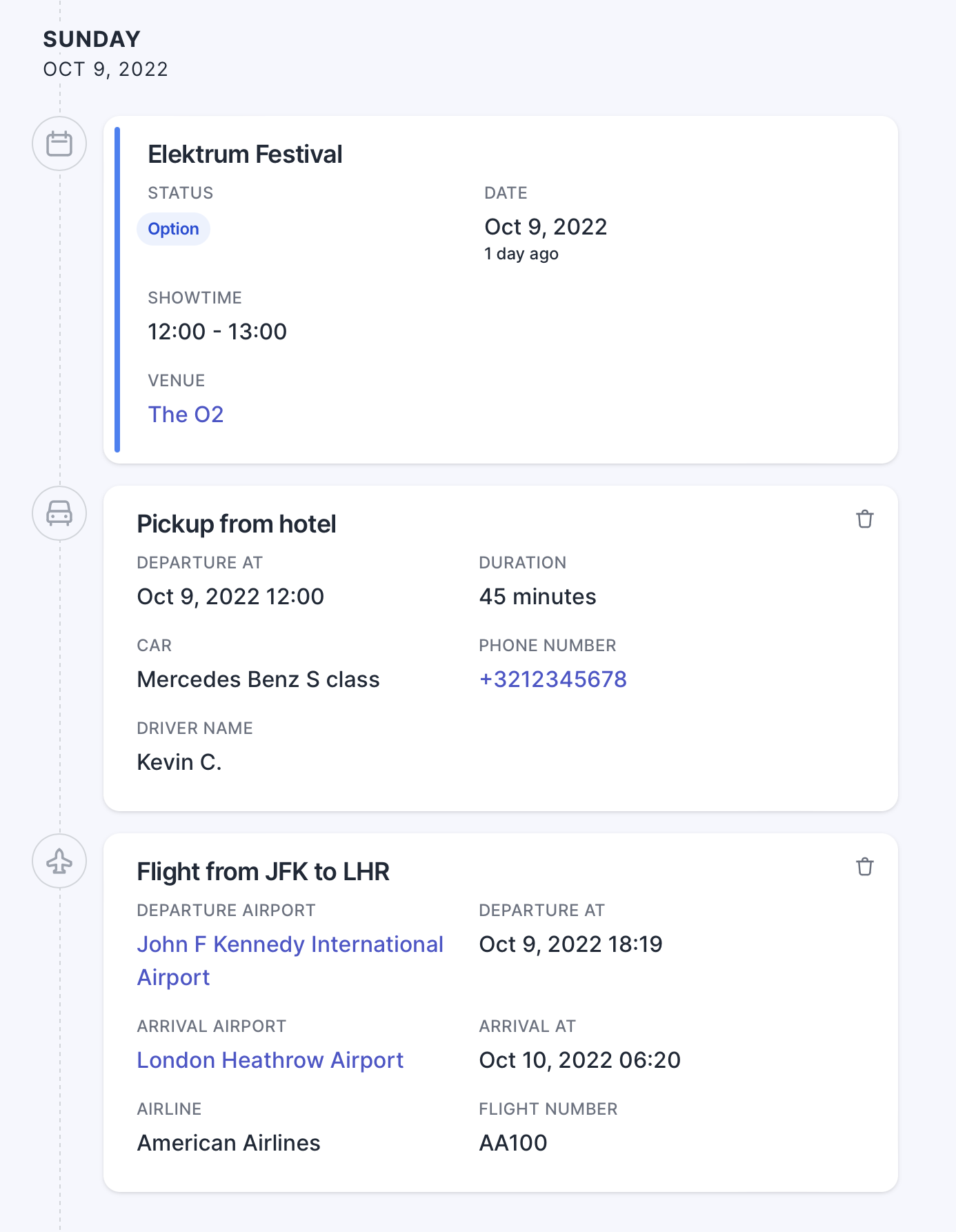The image details a comprehensive itinerary for an individual scheduled for Sunday, October 9, 2022. The itinerary begins with attendance at the Electrum Festival, which is set to take place from 12:00 to 13:00 at The O2. This is followed by a pick-up from their hotel, with the journey expected to last 45 minutes in a Mercedes Benz S-Class driven by Kevin C. The final item on the agenda is an international flight from John F. Kennedy International Airport (JFK) to London Heathrow Airport (LHR). The departure is from JFK on American Airlines flight AA100, scheduled to arrive in London on October 10th. The image succinctly captures the sequence of events, providing a clear and detailed view of the individual's planned activities and travel arrangements.